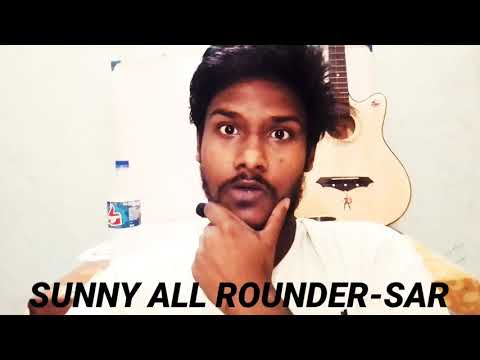This image is a thumbnail or screen grab from a social media video, possibly on YouTube, featuring a young man of likely Indian descent in his 20s. He has dark brown skin, black straight hair, and a black beard and mustache. He is wearing a white shirt and is seated in a chair. The man is positioned centrally in the image, looking directly at the camera with a surprised and inquisitive expression, resting his chin on his hand. Behind him, on his right, a white acoustic guitar hangs on a flat white wall, while to his left, there is a small plastic water bottle. Black bars frame the top and bottom of the picture, with bold black text at the bottom reading "SUNNYALLROUNDER-SAR." This text is possibly in a different language, adding contextual intrigue to the scene.